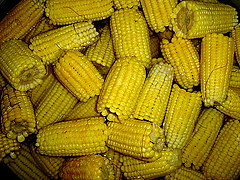The image is a small, rectangular photograph depicting a bright yellow pile of dried field corn cobs, many of which have been broken or cut in half. The arrangement of the corn is irregular, and the cobs are stacked atop one another, creating an impression of abundance. Some pieces of corn display dark strands of silk, and a few have tinges of either orange or red, especially towards the bottom of the pile. The corners of the image are darkly shaded, making it difficult to discern the surface on which the corn rests. This type of corn, which appears dry and tough, is typically intended for animal feed rather than human consumption and can be used in squirrel feeders. Lastly, there are noticeable dark shadows within the pile, highlighting the depth of the irregular stack.